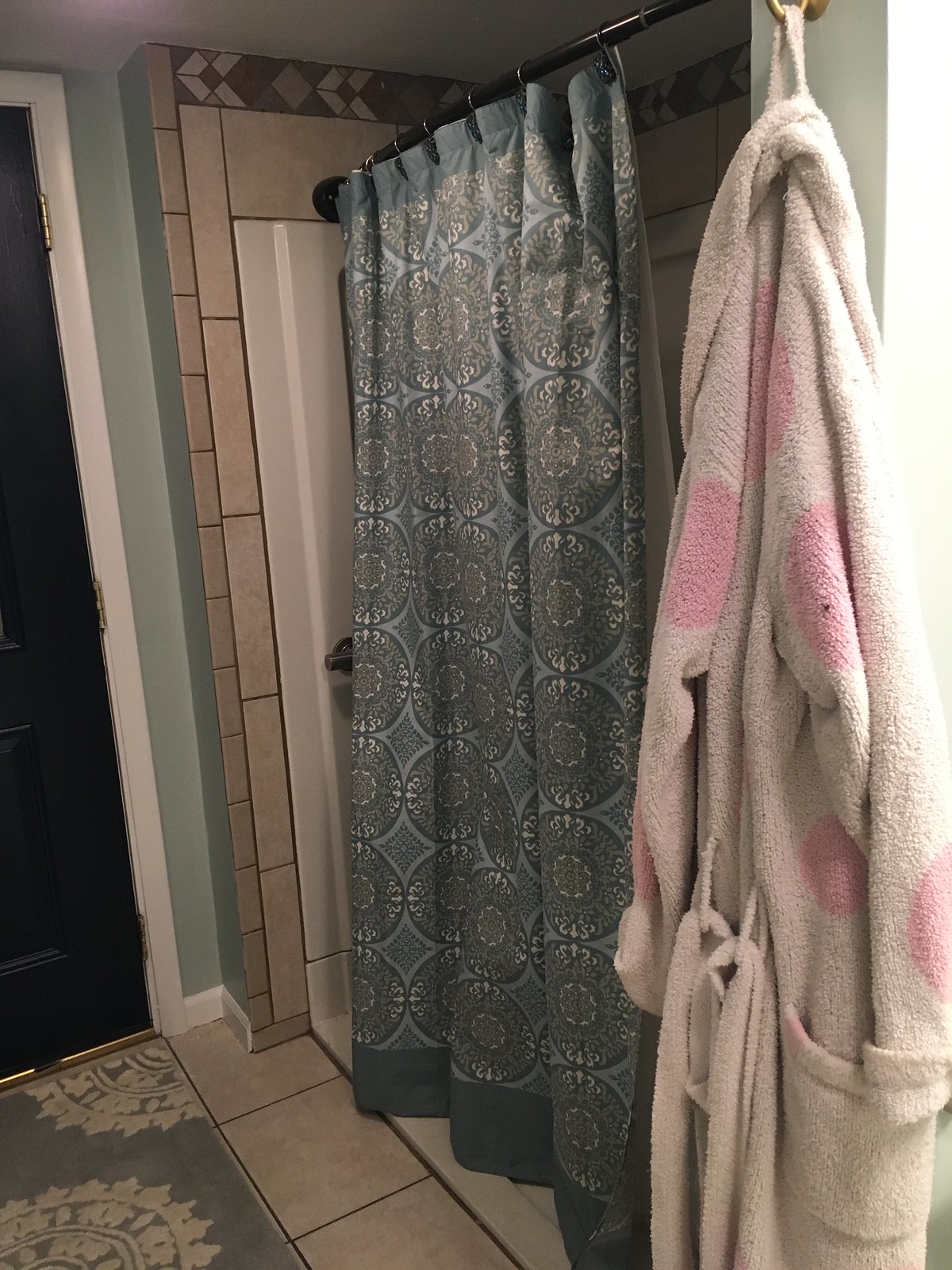The color photograph depicts a corner of a bathroom featuring a shower cubicle partially enclosed by a decorative shower curtain. The aquamarine shower curtain, adorned with intricate circular patterns, is suspended from a black metal rod affixed with metal hoops. Though the shower itself isn't visible, the ceramic tile walls and floor of the cubicle are evident. Adjacent to the shower, a predominantly white bathrobe with pink accents hangs from a hook. The room includes a thin, gray carpet with a white pattern, leading to a very dark brown door. Additionally, light brown tiles with a darker brown pattern adorn the upper section of the shower area, complementing the bathroom’s muted color palette.